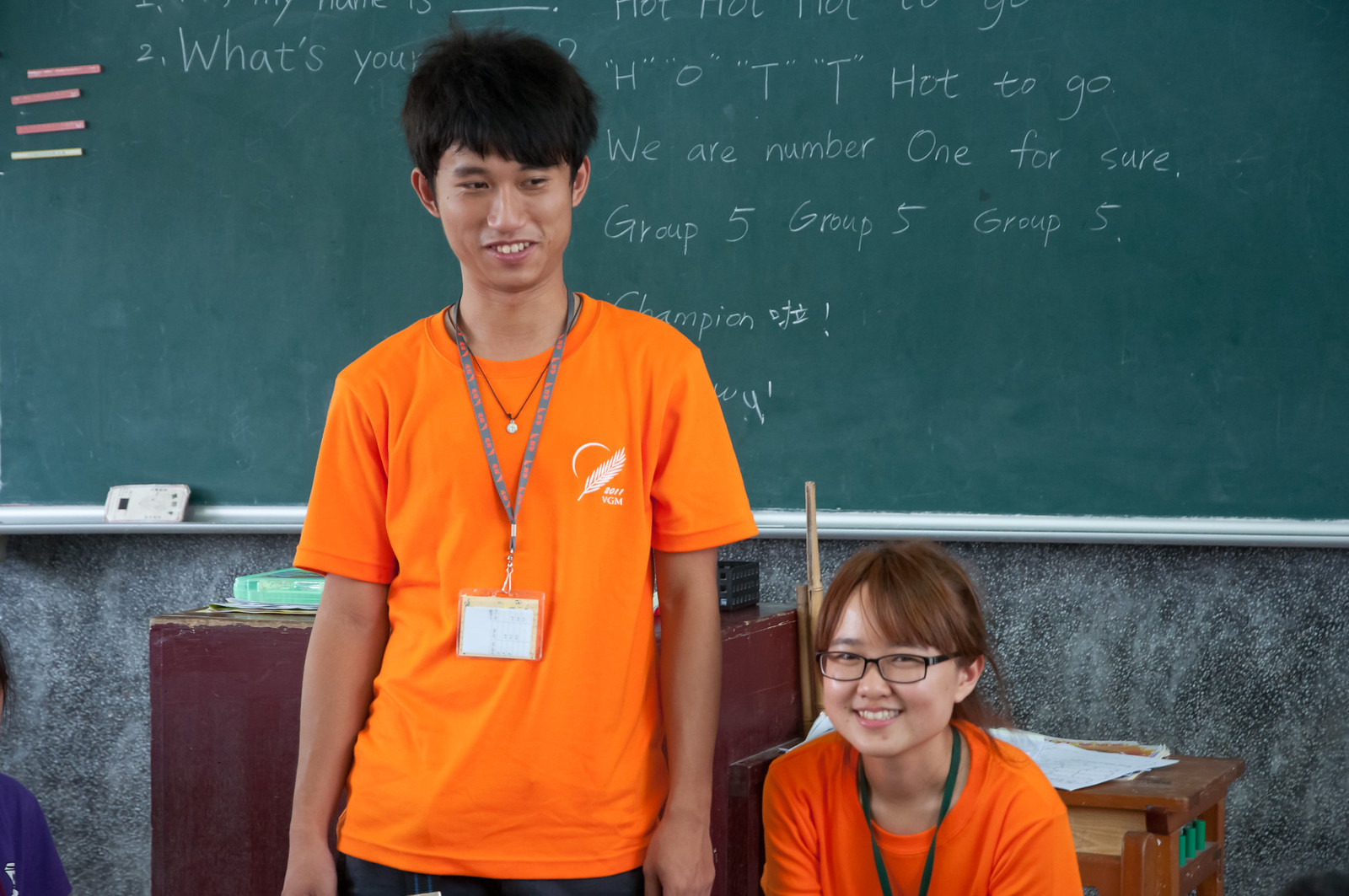In a classroom setting, this photograph captures two teenagers standing in front of a green chalkboard covered with handwritten messages that read, "What's your H-O-T-T hot to go? We are number one for sure. Group five, group five, group five, champion." Both students are wearing short-sleeve orange shirts with lanyards around their necks. The boy, standing on the left, has short, dark, fluffy hair and appears to be gazing slightly downward with a smile. He has a white plastic tag on his lanyard that rests at his abdominal level. The girl, on the right, has her red hair pulled back into a ponytail and wears black-rimmed rectangular glasses. She too is smiling. Behind the students are two desks; one holds various items including a pointer, and the other is smaller with some papers on it. An additional person, partially visible, is seated at the second desk.